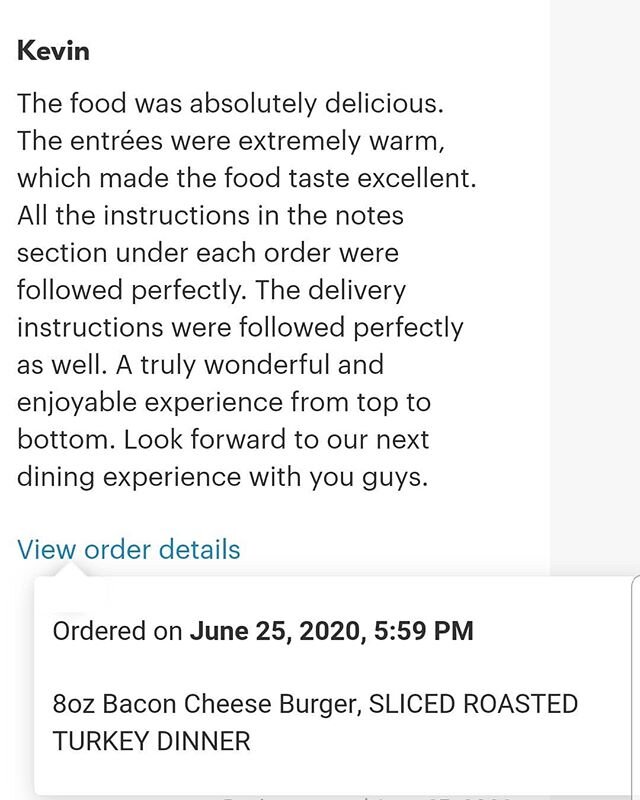**Detailed Caption:**

This vertical rectangular image features a detailed food review by Kevin at the top. In bold black lettering, his name "Kevin" is displayed prominently. Below Kevin's name, in regular black font, the review reads: "The food was absolutely delicious. The entrees were extremely warm, which made the food taste excellent. All the instructions in the notes section were followed perfectly. The delivery instructions were followed perfectly as well. A truly wonderful and enjoyable experience from top to bottom. Look forward to our next dining experience with you guys."

Under this review, in turquoise font, there is a clickable text saying "View Order Details." Extending from this clickable text, a white rectangular area appears horizontally. Within this area, in black font, it says "Ordered on," followed by bold black font indicating the date and time: "June 25, 2020, 5:59 PM." Directly below this in regular black font, it lists the items ordered: "8 oz Bacon Cheeseburger," with each letter capitalized, followed by "SLICED ROASTED TURKEY DINNER" in all capital letters.